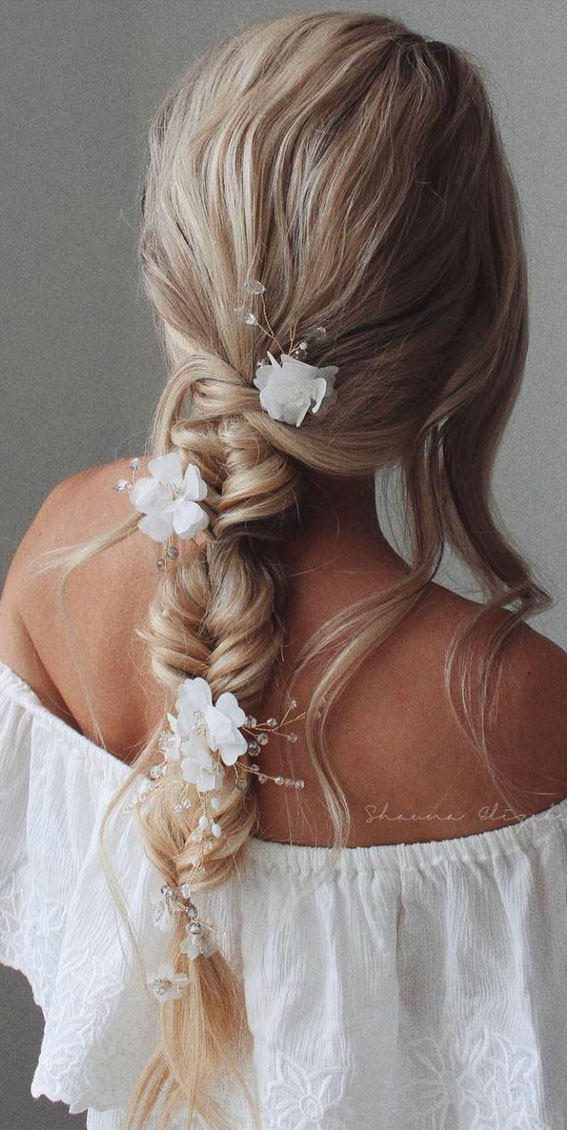This close-up angled image captures the elegant hairstyle of a woman with her back turned to the camera. She boasts long blonde hair accented with darker blonde to brown highlights, styled into a loose and intricate fishtail braid. Interwoven within the braid are three large white flowers reminiscent of plumerias, with smaller white blossoms adorning the lower part of the braid. Her bronze skin provides a striking contrast against her flowing locks, with soft, curled tendrils cascading over her right shoulder and a single tendril framing her left. She is dressed in an off-the-shoulder white blouse adorned with floral appliques and lace detailing. The background is a simple gray wall, ensuring all attention remains on her sophisticated look. In the right corner of the image, a watermark bearing the hair artist's name subtly signifies the creator of this hairstyle.